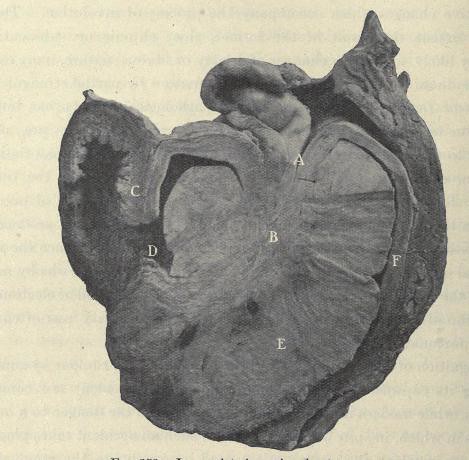In the image, there is a detailed model of a human heart, shaped distinctly like the actual organ. The model is grey and set against a yellow background, through which faint text can be seen, suggesting it may be an old photograph or an image of a printed page. The heart is cut open, revealing labeled sections corresponding to the heart's structure: 'CD' on the left side, 'ABE' down the middle, and 'F' on the right side. The exterior is bumpy, with a pointy part at the top that resembles an artery connection point. The left side shows a hollow area between the 'C' and 'D' labels, indicative of some internal cavity like an artery or valve. The photo has a weathered look, adding to its vintage feel.